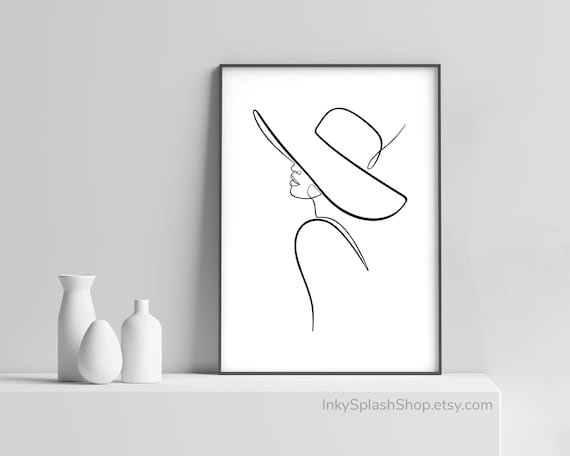The image portrays a serene and minimalist scene featuring a white wall and a smooth, concrete-like white shelf. On the left side of the shelf, there is a tasteful arrangement of three creamy white pottery pieces. The first piece is tall and egg-shaped with its pointed end up, the second is a flask-like vessel with a tapering neck reminiscent of an old milk jar, and the third is a wider, oblong bottle with a flared open top, somewhat akin to a modern molasses or beer bottle. 

To the right of these pottery items hangs a framed drawing, presented with a black frame against a white background. This simple and elegant line drawing depicts the partial profile of a woman, capturing her nose, lips, and a hint of her shoulder. The woman is adorned with a large, floppy hat that envelops her head, crafted with a single continuous line that adds a touch of sophistication and mystery. Below the artwork, the inscription "inkysplashshop.etsy.com" suggests that the drawing is available for purchase from this online store. The composition of pottery and drawing evokes a sense of quiet elegance and refined simplicity.